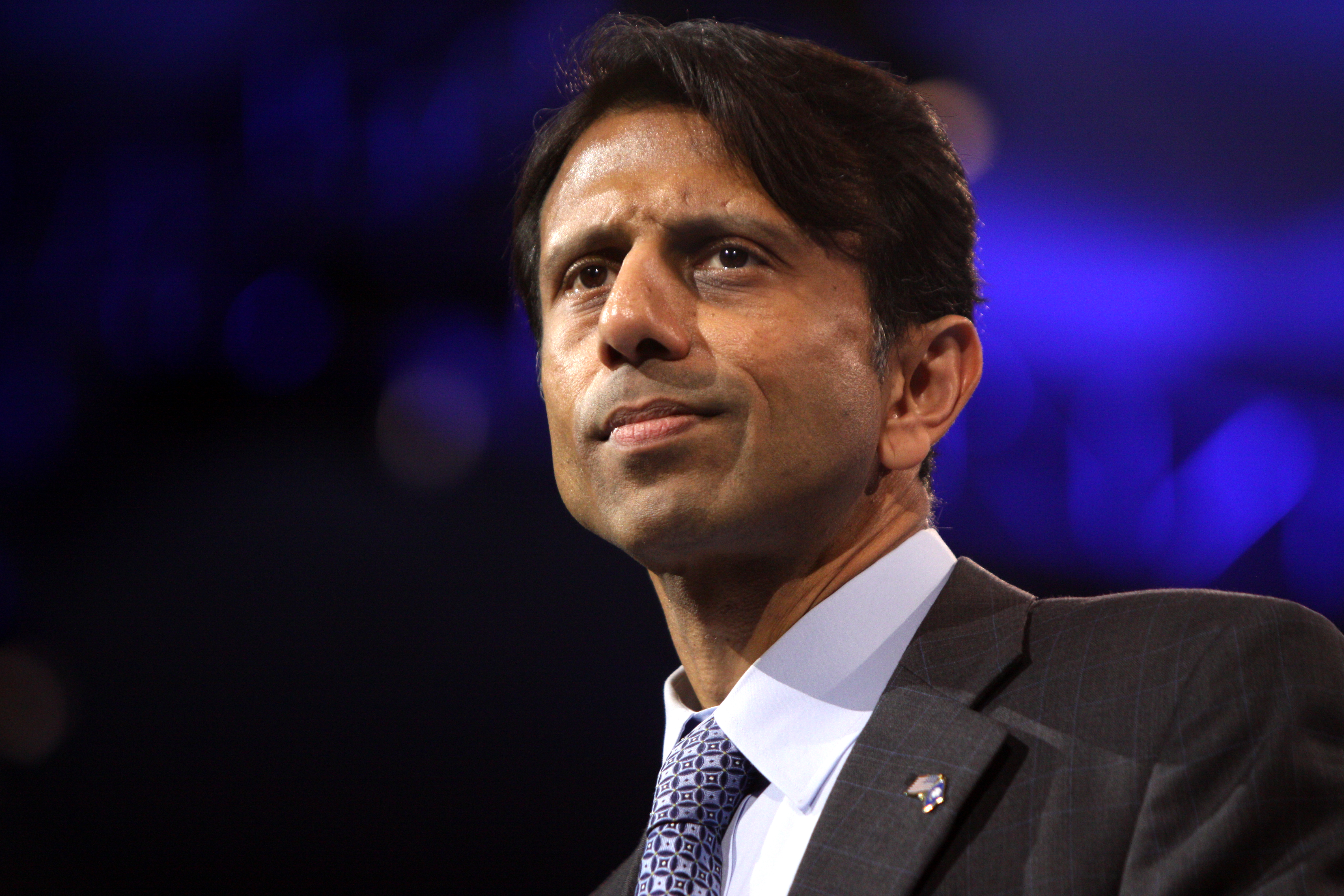The image portrays a close-up of an Indian man who resembles Bobby Jindal. He has dark caramel-colored skin, short black hair, and brown eyes. His facial expression appears concerned and unhappy, as if he's deep in thought or feeling frustrated. The man is dressed in a dark charcoal gray suit with checkered pinstripes, a white collared shirt, and a tie that features a pattern of small squares. A metallic lapel pin decorates the right side of his suit jacket collar. The background highlights a contrast with a bluish-purple light focusing on the upper right corner, while the lower-left corner remains darker with a black backdrop, adding a shadowy effect over the man. The context suggests he's speaking at some sort of event.